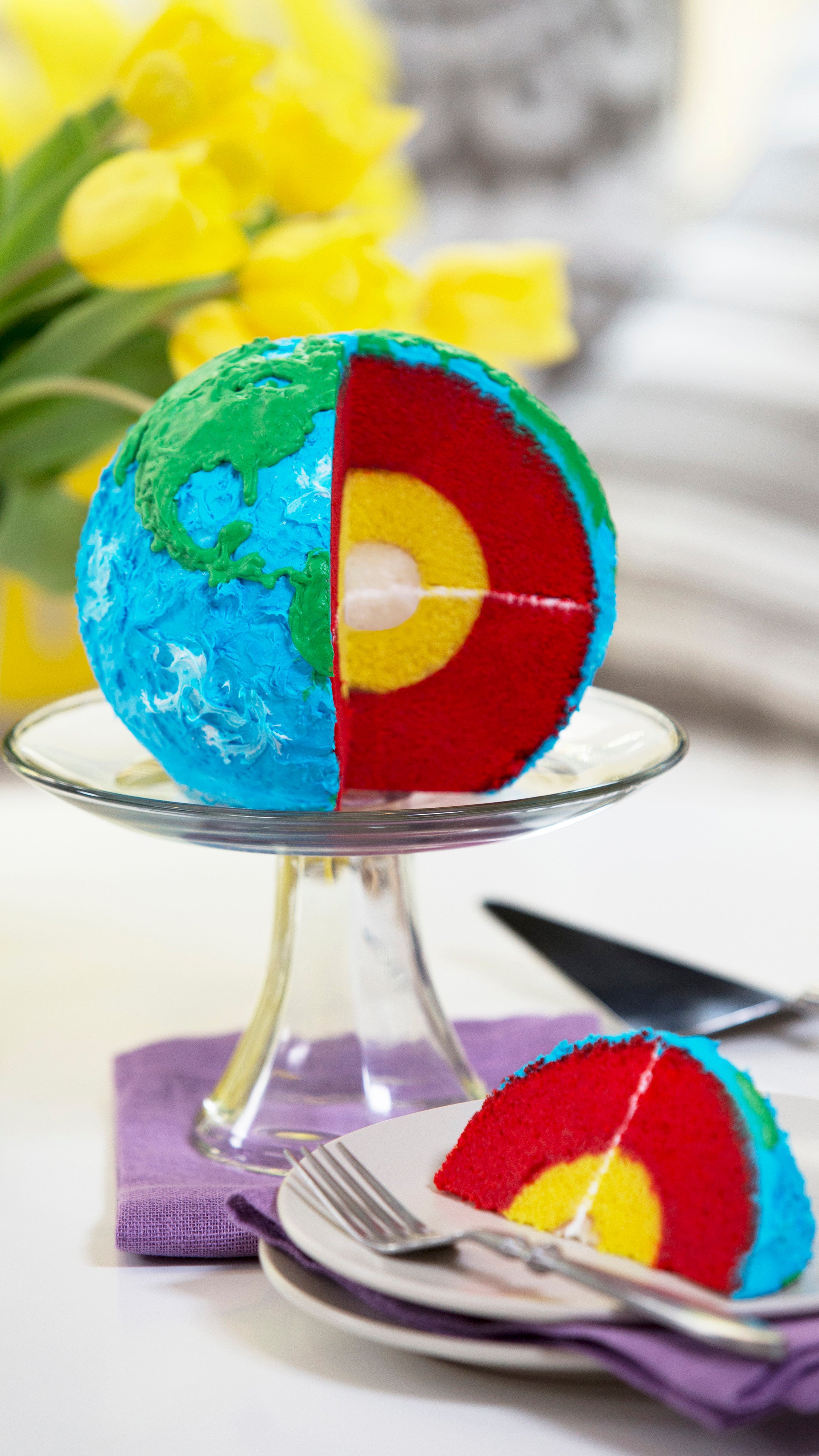This close-up, vertically-aligned photographic image, taken indoors, captures an intricately designed cake that resembles a globe, complete with a detailed map of Earth. The cake, expertly frosted to highlight the blue Atlantic Ocean, North America, Central America, and parts of South America, is seated on a glass cake platter with a round base, placed on a purple tablecloth. A slice of the globe-shaped cake has been cut out and laid on a white china plate, which rests atop a purple napkin and another plate. The interior of the cake mimics the Earth's layers, featuring concentric circles in red, orange, and a white center, reminiscent of the Earth's core. Accompanying the plate is a fork, and to the right, a cake spatula; meanwhile, the upper left-hand corner of the image showcases an out-of-focus bouquet of yellow tulips. The background remains blurry, putting the meticulously crafted cake and its slice at the forefront of this striking image.